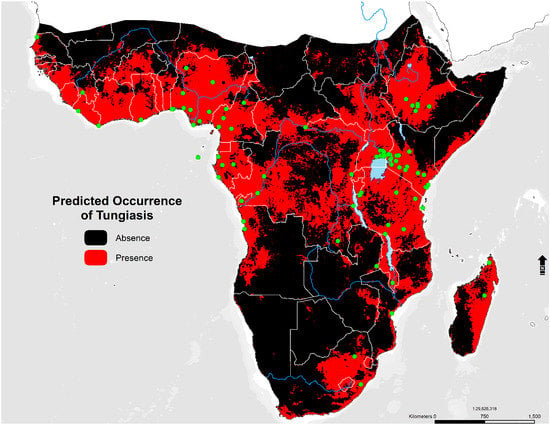This is an image of a map of Africa. The map displays boundaries of nations with white lines, and rivers are illustrated with blue lines. The majority of the map is divided into regions colored in black and red. The central portion predominantly shows red, indicating the presence of a factor referred to in the key on the left side of the map, titled "Predicted Occurrence of Tungiasis," a disease. The upper and lower regions are marked in black, indicating an absence of the condition. Madagascar is uniquely colored, with half in black and half in red. Scattered throughout the map are green dots, though the key does not explain their significance. The surrounding oceans are depicted in light gray. On the bottom right side of the map, there is a long rectangle, possibly for reference measurements.